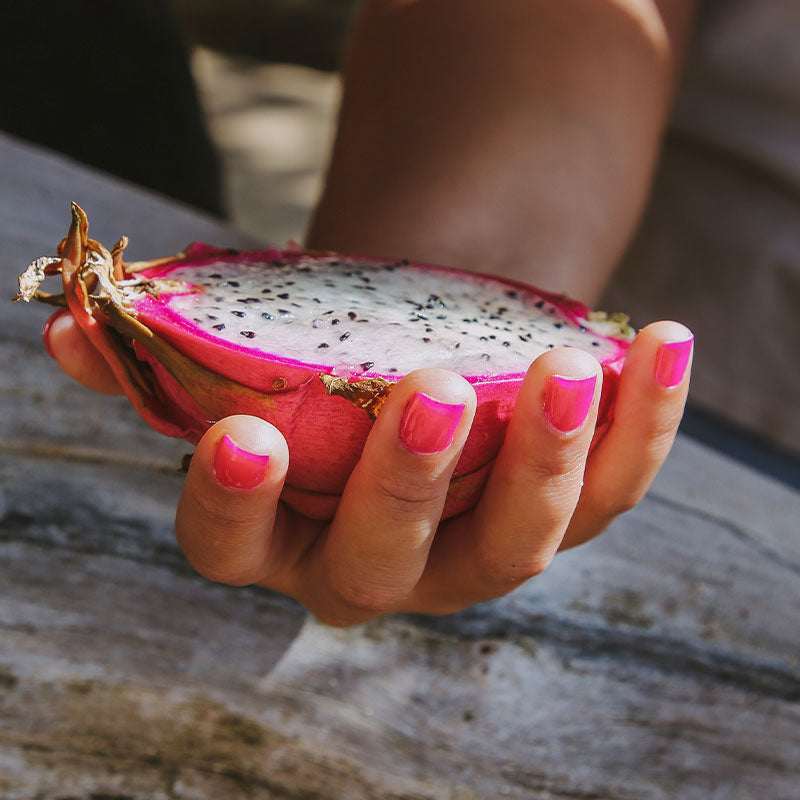The image depicts an outstretched hand, likely belonging to a female with neatly manicured pink fingernails, holding half of a dragonfruit. The hand is positioned palm-up towards the camera, displaying all fingers except the thumb. The vibrant pink skin of the dragonfruit matches the color of the manicured nails. The fruit is cut open, revealing its white, fleshy interior dotted with tiny black seeds. At the thumb area, a bit of the dragonfruit's dry stem is visible. The background appears to be an outdoor scene with what seems to be a surface made of either rock or a worn wooden table featuring gray, brown, and white tones, slightly blurred in the image.